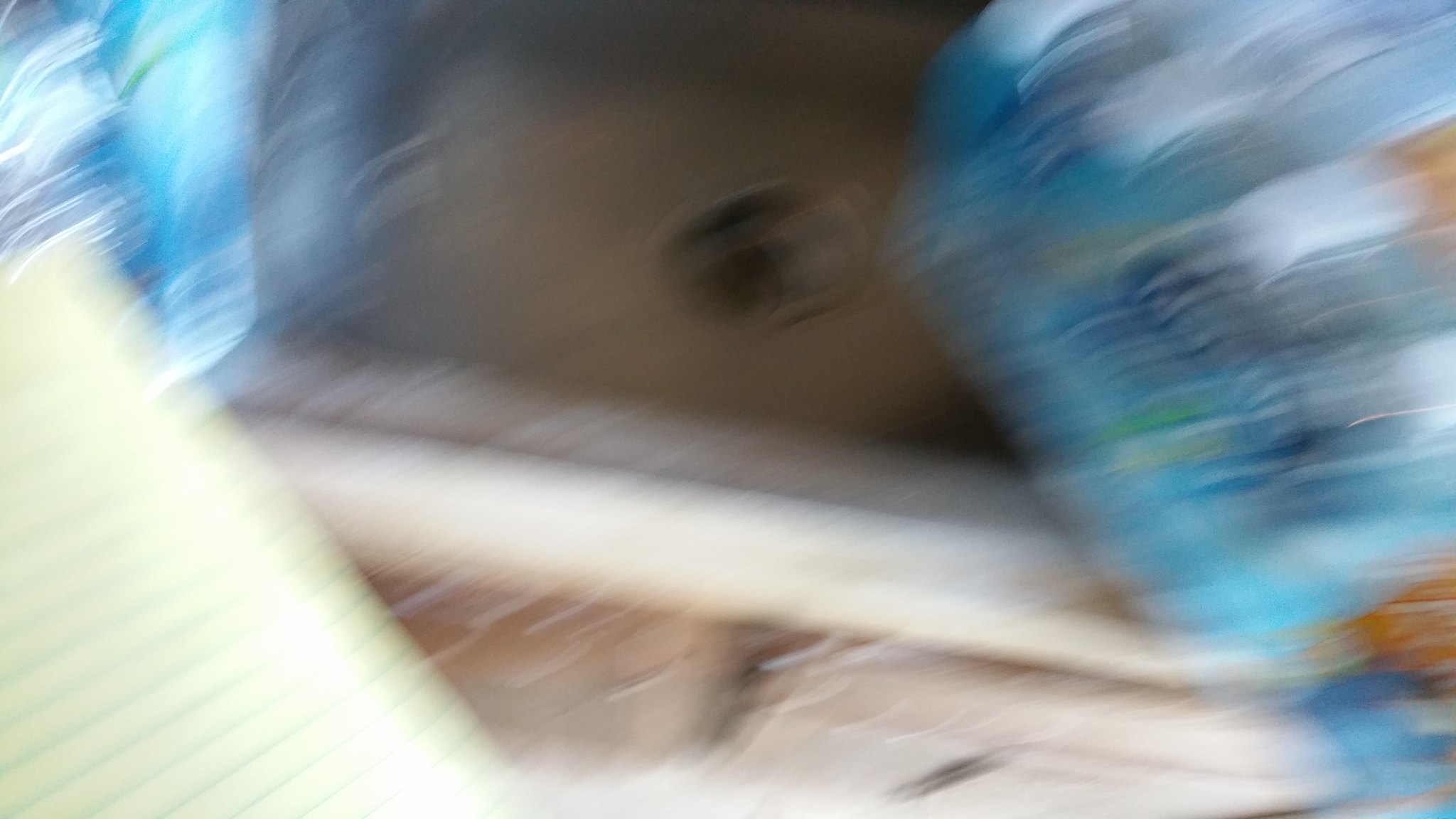This photograph presents a large, rectangular layout, but is notably blurry and out of focus. In the background at the top, a silver kitchen sink is faintly discernible, complete with a round central drain integrated into the countertop. The countertop, appearing to be white, borders the sink but remains indistinct due to the lack of clarity in the image. On the right edge of the sink, a case of bottled water with blue plastic packaging is partially visible, displaying the white caps of the bottles from above. Similarly, on the left edge of the sink, the corner of another water case peeks into the frame. The bottom left corner features a white piece of paper, possibly a list or a book page, with black text running down its length, angled slightly within the composition.